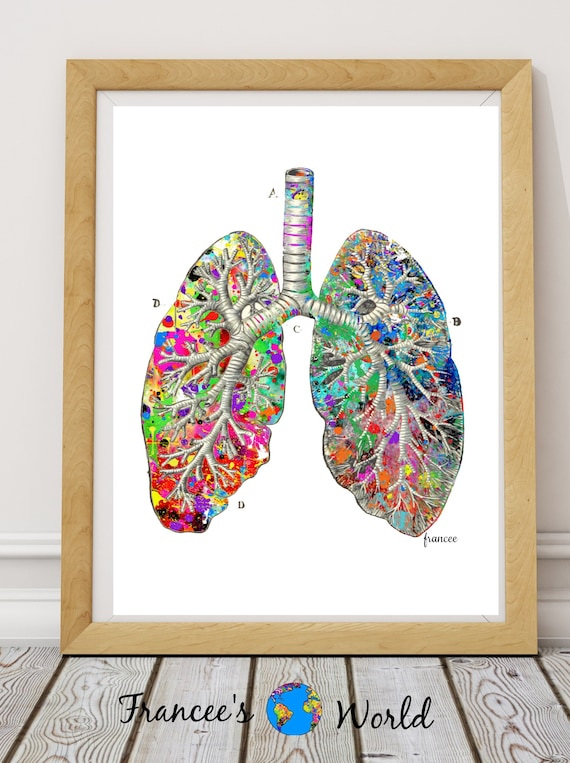This image features a framed artwork leaning against a white wall with a baseboard, positioned on a wooden floor. The frame is made of tan wood and contains an illustration of a pair of human lungs. The illustration showcases a vibrant, colorful array akin to a splatter paint style, with hues of pink, green, yellow, blue, dark blue, orange, black, and white. The pulmonary tubes branching into the lungs are shaded in gray, adding a ribbed texture to the design. Each section of the lungs is labeled with letters A, B, C, and D, with D repeating in two areas. Below the lungs, the name "Francie" is written. Beneath the framed illustration, black lettering spells out “Francie’s World,” with a small globe icon situated between the words "Francie’s" and "World." The cursive text and playful colors contribute to the unique and eye-catching aesthetic of the piece.